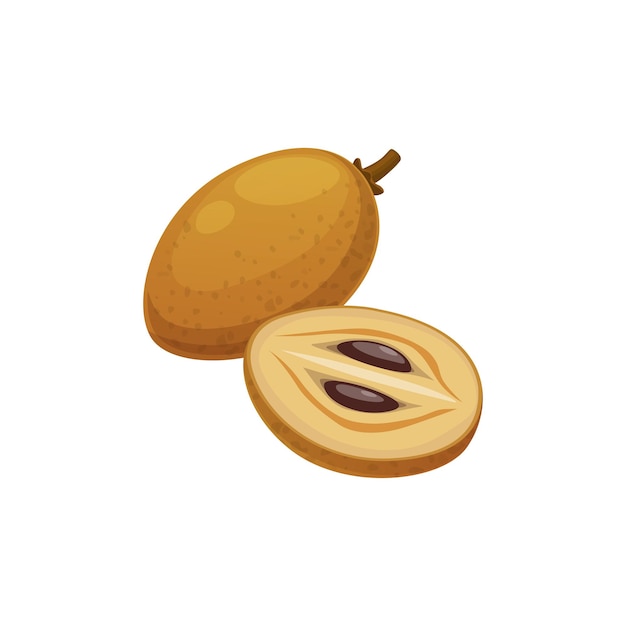This illustration showcases an oblong-shaped, orangey-yellow fruit with a small brown stem, set against a plain white background. The fruit's exterior is speckled and darker in color, resembling a peach or an olive, but its exact type is ambiguous. In the foreground, a longitudinal slice of the fruit reveals its interior. The inner flesh is a light beige, almost off-white, accented by a central white stripe and flanked by two large, brown, slit-like seeds. The detailed depiction indicates the fruit to be a kind of stone fruit, though its precise identity remains unclear.